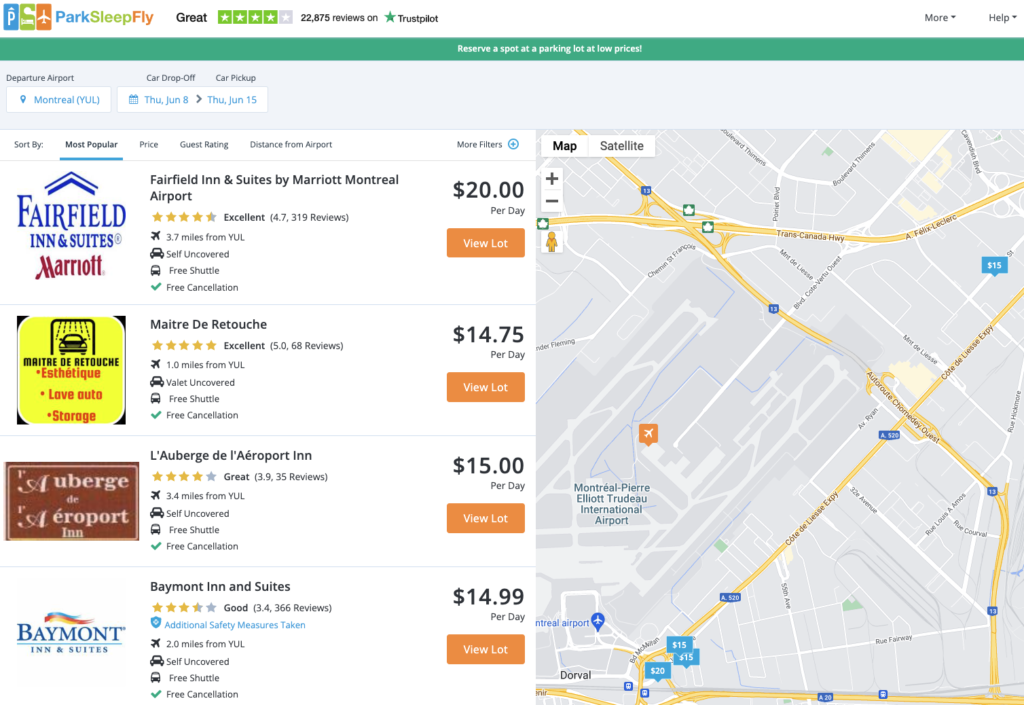This is a detailed screenshot of the "Park Sleep Fly" website, featuring its distinctive logo at the top left—comprised of the stylized letters "PS" and an airplane shape forming part of the letter "F". The words "Park" in blue, "Sleep" in green, and "Fly" in orange are prominently displayed.

The screenshot shows the "Most Popular" tab selected, indicating that users are viewing the top-rated options. At the top, a 4-star rating is visible, accompanied by 22,875 Trustpilot reviews, suggesting a high level of customer satisfaction. In the top-right corner, there are "More" and "Help" buttons with dropdown menus for further navigation.

Just below, a green bar invites users to "Reserve a spot at a parking lot at low prices," emphasizing affordability. Filters applied include Montreal (YUL) as the departure airport, with a car drop-off on Thursday, June 8th, and car pickup on Thursday, June 15th.

Users can sort the results by "Most Popular," "Price," "Guest Rating," and "Distance from Airport," with "Most Popular" currently selected. The main section displays various suites and inns, each with their per-day pricing clearly listed. A prominent orange "View Lot" button next to each option allows users to get detailed information about each listing. An embedded map on the right helps users visualize the locations of the parking options. This comprehensive view helps travelers find the best parking, hotel, and shuttle deals for their trips.